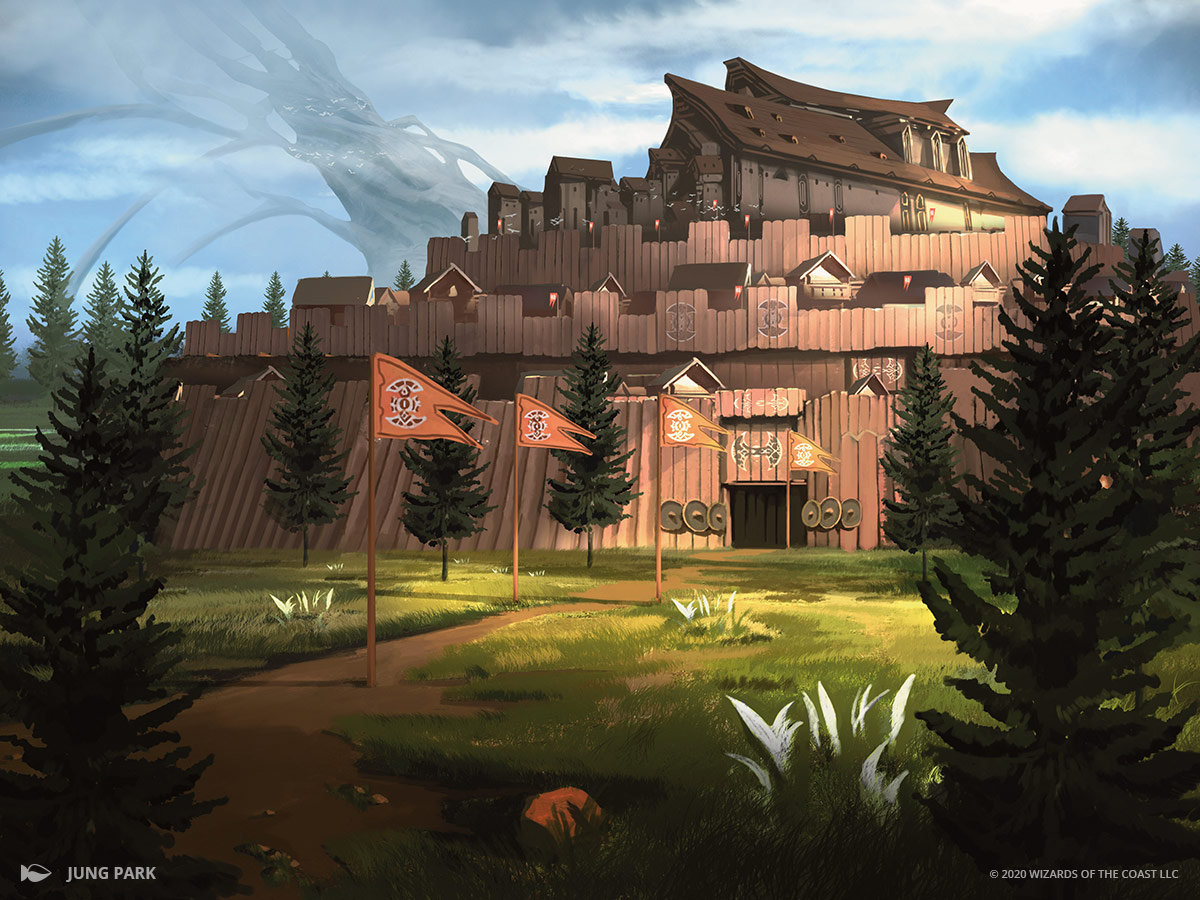This detailed scene showcases a digital rendering from a video game, depicting an Asian-inspired fortress or tower complex enclosed within tiered, reinforced wooden walls, creating a gated area. The main structure has a brown roof and tan-colored siding, and it's surrounded by a mix of smaller buildings. The setting features a dirt pathway leading up to the gate, lined with orange flags displaying clan or tribal insignias. The landscape includes evergreen and pine trees, with a notable, giant tree-like structure rising in the distant horizon. The sky is blue with some clouds, adding depth to the scene. In the lower corners, the image credits 2006 Wizards of the Coast LLC and the artist Jung Park, along with a small fish symbol.